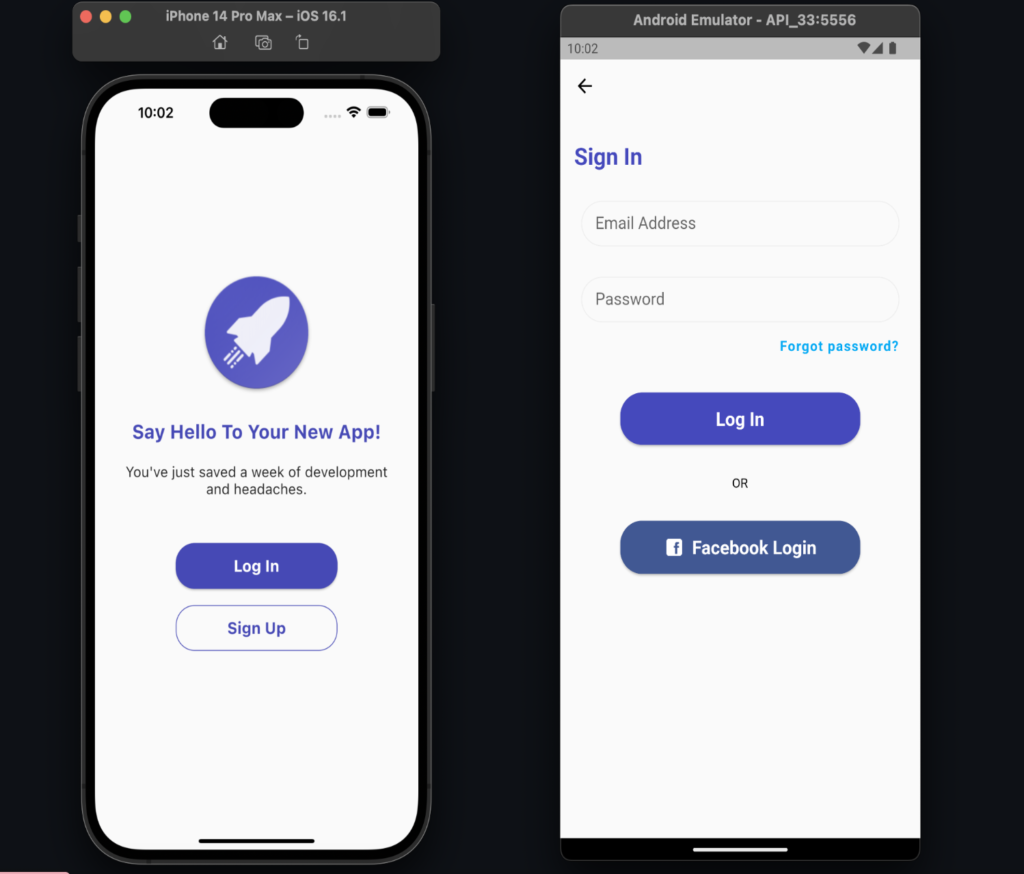In this image, we are presented with a screenshot framed against a solid black background. The focus is on a black cell phone displayed to the left. The phone's screen is active, showcasing a white background. In the upper left corner, the time is displayed as "10:02" in black text. The upper right corner indicates a full battery and active Wi-Fi connection. Centered on the screen is a periwinkle circle containing a white space rocket icon. Beneath this icon, periwinkle text reads, "Say hello to your new app. You've just saved a week of development and headaches." Below this text, there is a periwinkle-colored "Login" button, followed by a white "Sign Up" button.

To the right of the phone, another screenshot features a sign-in interface for an app. It includes fields for entering an email address and password, accompanied by a blue "Login" button. Underneath the login button, there is an option to log in with Facebook. Above the login section, small blue text reads, "Forgot password?"